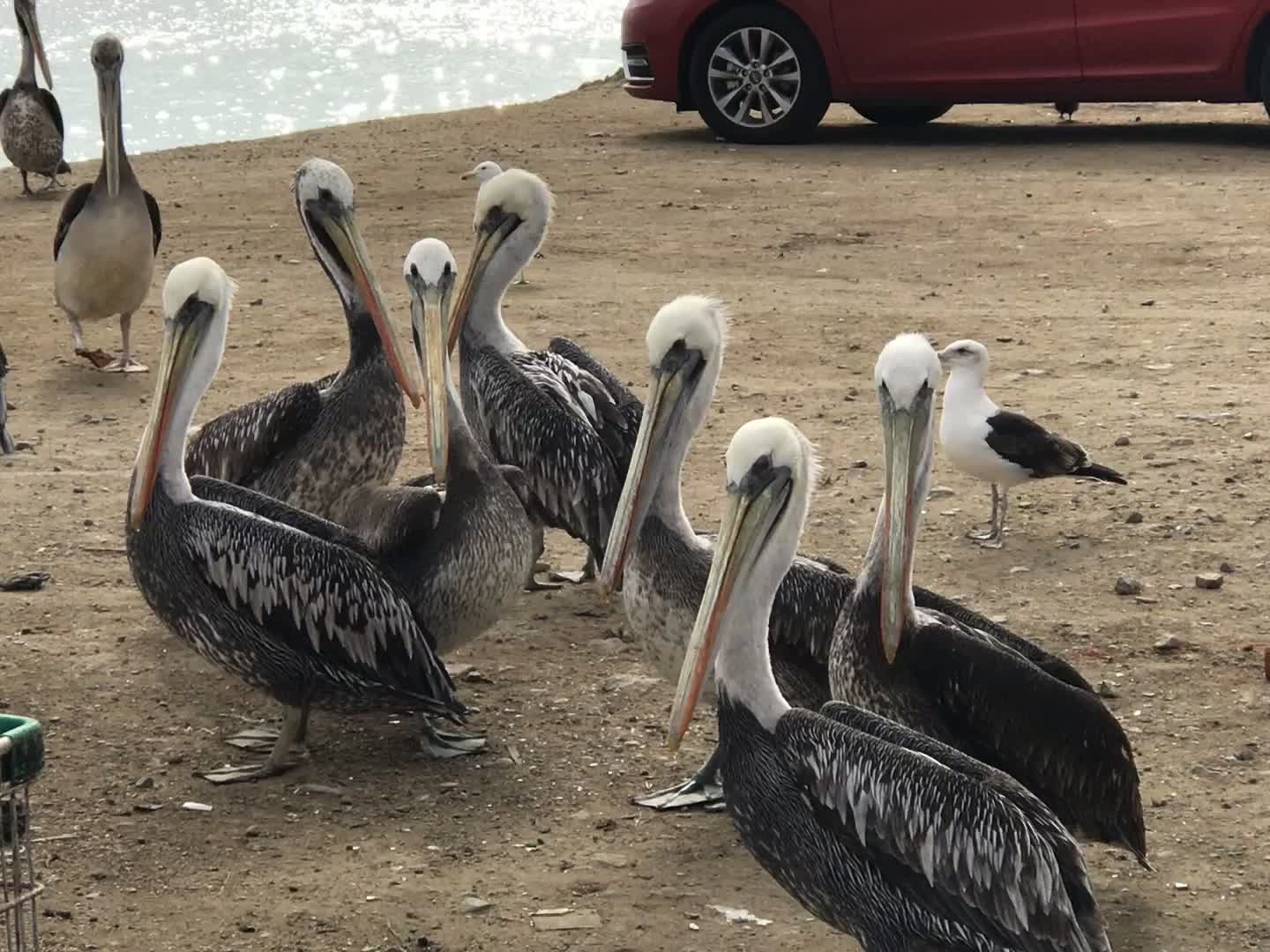The outdoor photograph captures a scene on a dirt area adjacent to a body of water, visible in the upper left-hand corner, shimmering under sunlight. In the upper right-hand corner, the lower portion of a red car with black tires is partially visible. Dominating the center of the image is a group of nine pelicans with brownish-gray bodies and long, slightly curved white necks. They have elongated brown beaks and are predominantly clustered together in the front middle part of the frame, totaling seven closely packed birds. Just behind the main group of pelicans stands a small pigeon or seagull with a white and gray coloration. The ground is a sandy dirt brown scattered with small gray rocks and a bit of litter.